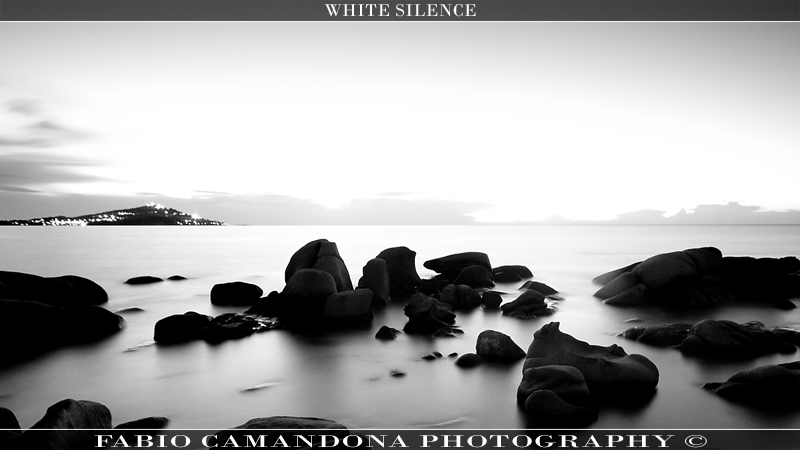This black and white photograph, resembling a scenic postcard, captures a tranquil bay scene by Fabio Kamandona Photography. In the foreground, a series of rocks protrude from a serene, almost smoky-looking body of water, which might be an effect of post-production editing. The background reveals a vast landmass adorned with sparkling lights, adding a touch of liveliness to the otherwise peaceful landscape. The image, labeled "White Silence" at the top and "Fabio Kamandona Photography Copyright" at the bottom, exudes a sense of calm and timeless beauty, perfectly suited for a postcard.